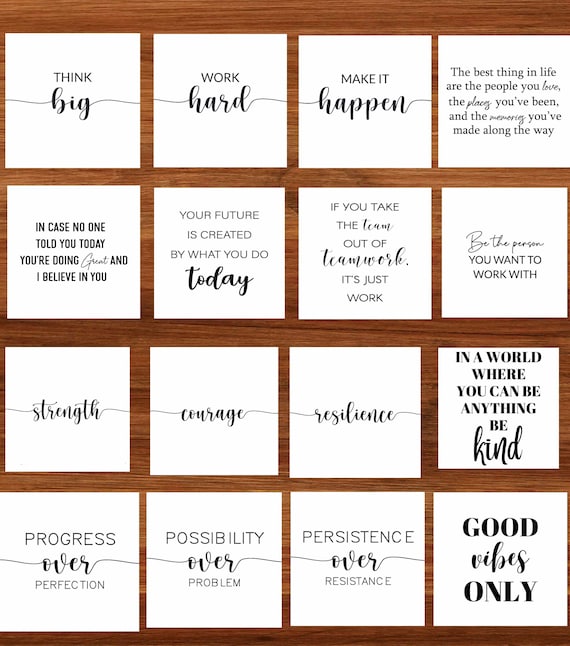The square image captures a meticulously arranged set of 16 white posters, each adorned with motivational phrases in black ink, set against a brown wooden surface with visible grains. The posters are laid out in four rows of four, each containing one or two lines of text in varying typographic styles. The phrases connect in a seamless flow, offering an array of uplifting messages such as "Think big," "Work hard," "Make it happen," and "The best things in life are the people you love, the places you've been, and the memories you've made along the way." Additional sentiments include "In case no one told you today, you're doing great and I believe in you," and "The future is created by what you do today." There's also a note on teamwork: "If you take the team out of teamwork, it's just work," alongside advice to "Be the person you want to work with." Other inspiring words include "Strength," "Courage," "Resilience," "In a world where you can be anything, be kind," "Progress over perfection," "Possibility over problem," "Persistence over resistance," and finishing with the cheerful "Good vibes only."